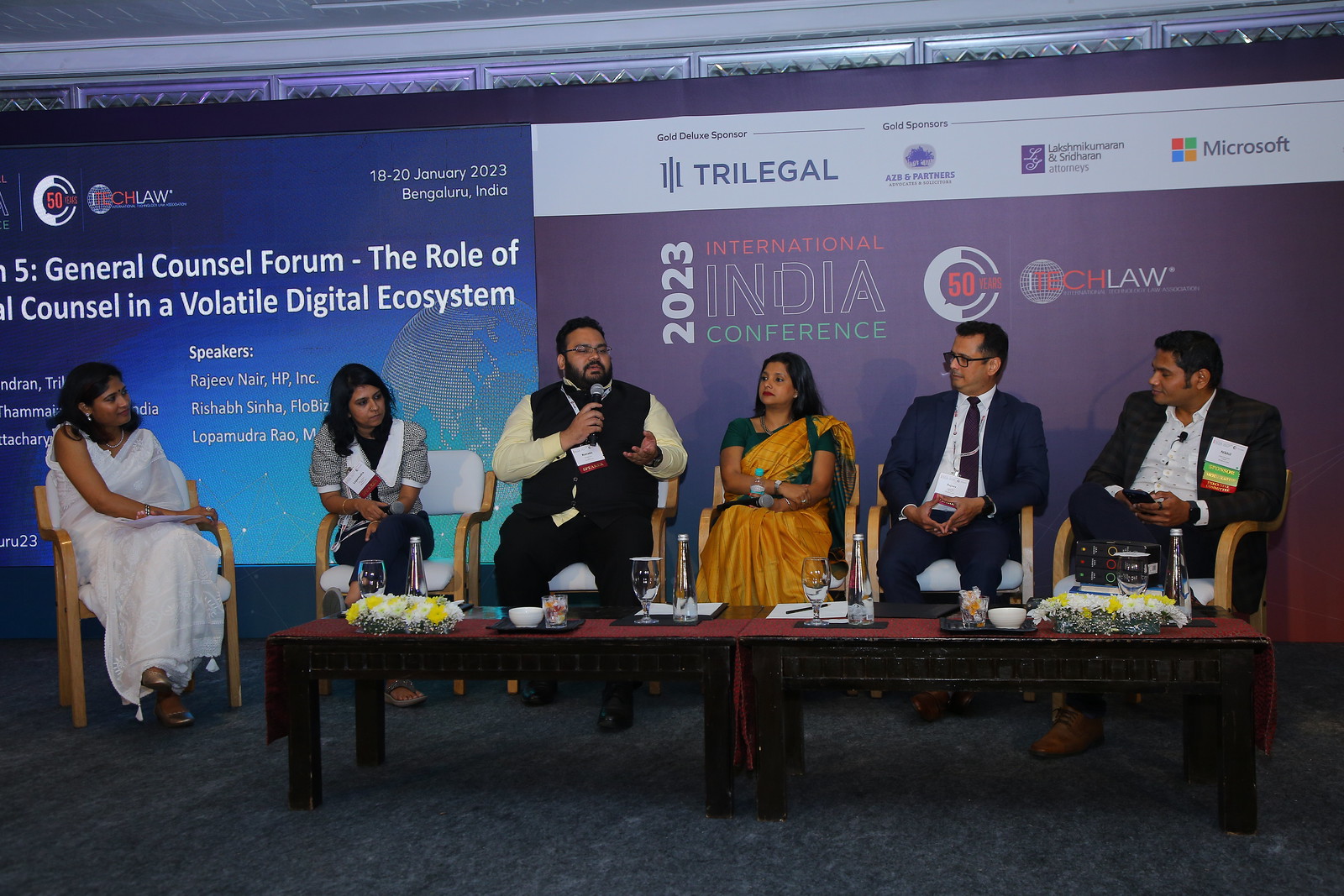The image captures a panel at the 2023 International India Conference, with seven individuals seated behind two low coffee tables arranged together. The backdrop features large bright monitors displaying the event's title along with sponsor logos like Trilegal and Microsoft. Central to the image is a man in the center holding a microphone in his right hand and wearing glasses, a black vest paired with a long-sleeved yellow shirt, and a lanyard with a white and red tag. Flanking him to his left is a woman in a gray and white blouse, and next to her, another woman in a white see-through one-piece dress. To his right is a woman in a green and gold dress with long dark hair, followed by a man in a dark suit with a white shirt, glasses, and hands steepled in front of him. Another man on the far right is dressed in a dark checked coat and white shirt. The panelists are adorned with name tags, indicating their roles as presenters at the conference. The table before them holds several water glasses and a few bowls, suggesting they might be in the midst of a discussion or Q&A session. Behind them, additional text on the monitors mentions "General Council Forum" and touches on the role of councils in a volatile digital ecosystem.